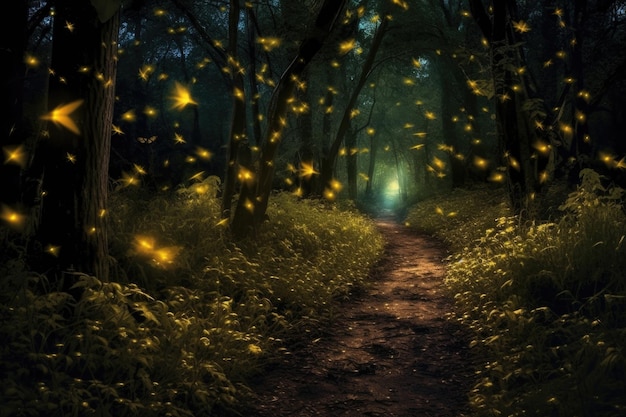The image depicts a digital graphic of a dark, nighttime forest with a central dirt path stretching from the foreground to the background. The forest is densely packed with tall trees on both sides, their branches and leaves forming a canopy that partially obscures the sky. Lush, overgrown grass in shades of yellow and light green lines both sides of the path. The forest is teeming with countless fireflies or possibly yellow butterflies, numbering in the hundreds, their lights creating a magical, glowing ambiance. At the end of the dirt path, a bright light source suggests an exit from the forest. Above the trees, a faint light blue sky or moonlight peeks through, adding a subtle illumination to the scene.